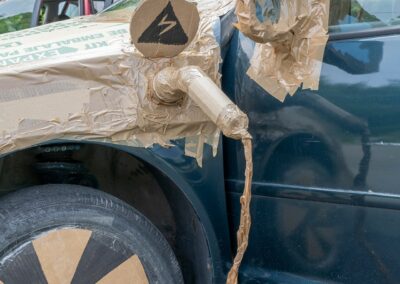The photograph depicts the front side of a dark blue or black vehicle, largely covered in brown packing tape and other makeshift materials. Prominently, the side view mirror and portions of the door and hood are enveloped in brown tape. The front wheel and coil springs are visible, with the wheel rim partially obscured by a piece of metal or cardboard painted in yellow and black triangular segments, resembling pizza slices. A notable feature is a taped construction on the hood that mimics a gas nozzle, with a long strip of tape extending from it, giving an illusion of pouring liquid. Above this taped 'nozzle,' there's a round piece of cardboard adorned with a triangle and a lightning bolt symbol, possibly indicating energy or fuel. The artistic yet chaotic use of tape and cardboard creates an abstract, almost surreal appearance on the vehicle.